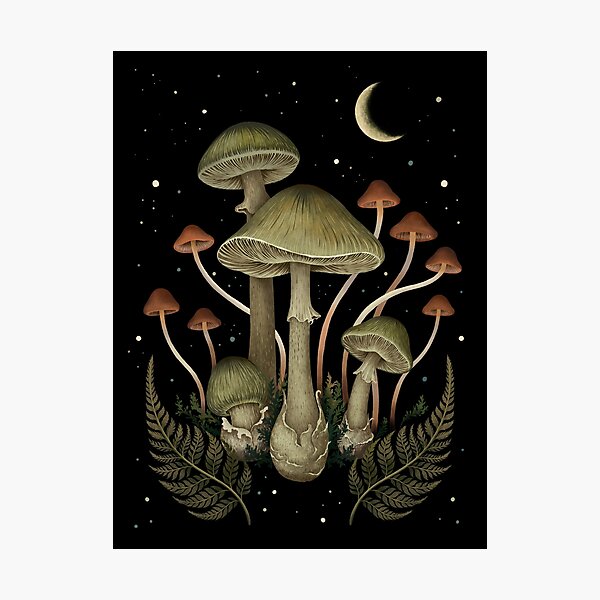This captivating painting features a surreal night scene with a black background, sprinkled with yellowish-white stars of varying sizes and a slightly yellow crescent moon positioned in the top right corner. Dominating the foreground is an intricate cluster of floating mushrooms. The central mushroom, near the bottom third of the image, displays a flaky beige bulb from which sprouts a light brown stem, topped with another beige segment, a flanged underside, and a slightly greenish-brown cap. Behind it to the left is a taller, similar mushroom with a more rounded cap, while a very short mushroom capped and with a small amount of stem sits at the bottom left. A shorter, angled version of the main mushroom tilts off to the right in the bottom-right corner. Complementing these earthy fungi are stringy pink and white gradient stems ending in red caps scattered in the background, flanked by curling gray-green leaves—one extending from the bottom left and looping upwards to the left, the other curling up to the right. The leaves, resembling fern fronds, frame the scene, evoking an ethereal quality as if everything is suspended in this magical, starry space.